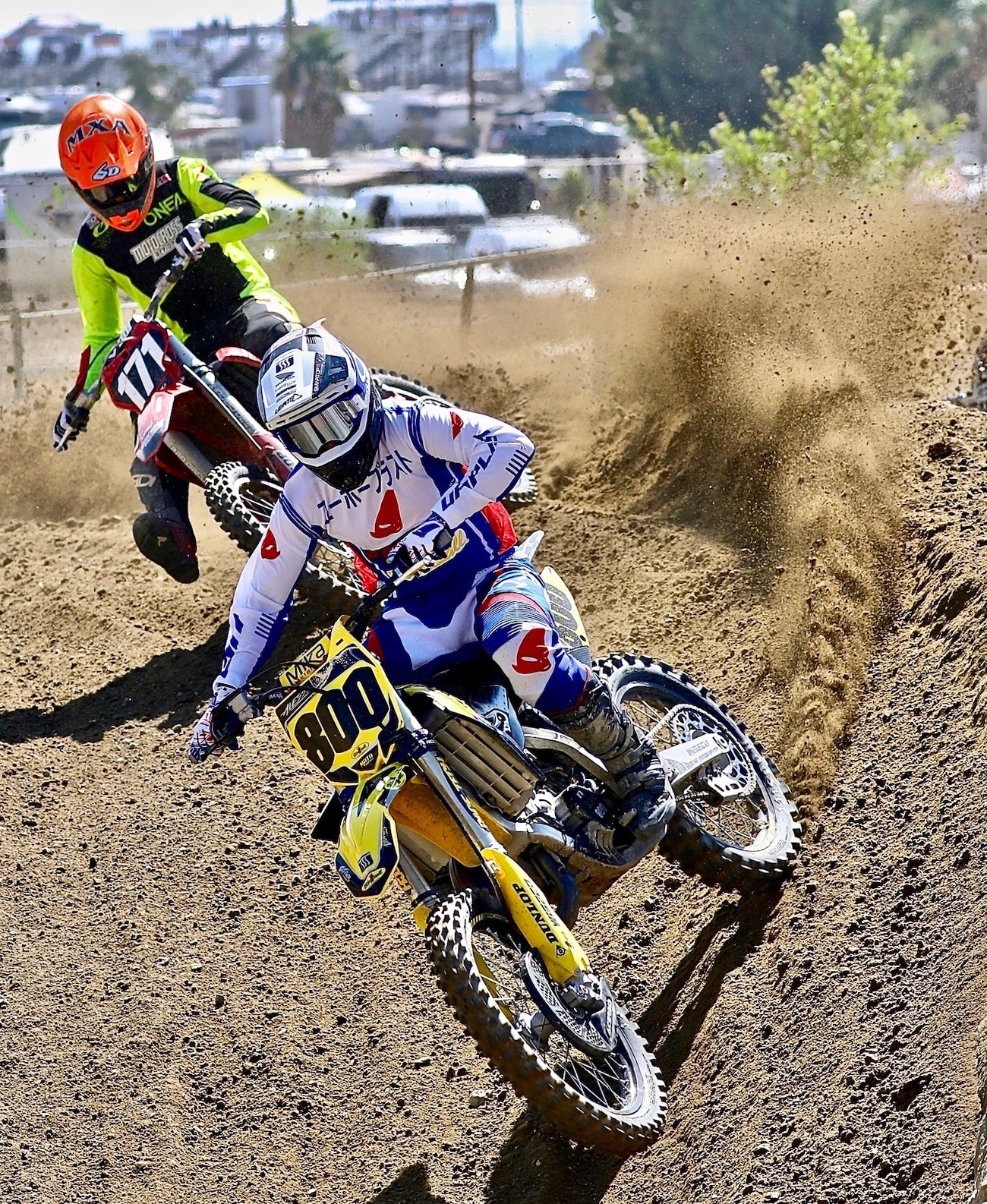In this captivating image, two death bikers are captured racing through a sandy dirt course, kicking up impressive clouds of dust. The biker leading the race, numbered 800, rides a predominantly yellow bike and is negotiating a bend with finesse. He dons a striking outfit in white, blue, and red, complemented by a blue and white helmet that features a black chin guard and reflective silver glasses. Notably, his uniform also has Japanese writing, adding a unique touch. Trailing behind is biker number 171, easily identifiable by his black and neon yellow jumpsuit and an unmistakable orange helmet marked with "MXA." His bike is primarily red, and he sports black glasses. Both riders are tilting slightly, with their right shoulders lower than their left, indicating the inclined terrain they are navigating. The background is a blurred mixture of white cars, resembling a parking lot, and buildings bordered by an aluminum gate-type fence, providing a stark contrast to the intense action in the foreground.